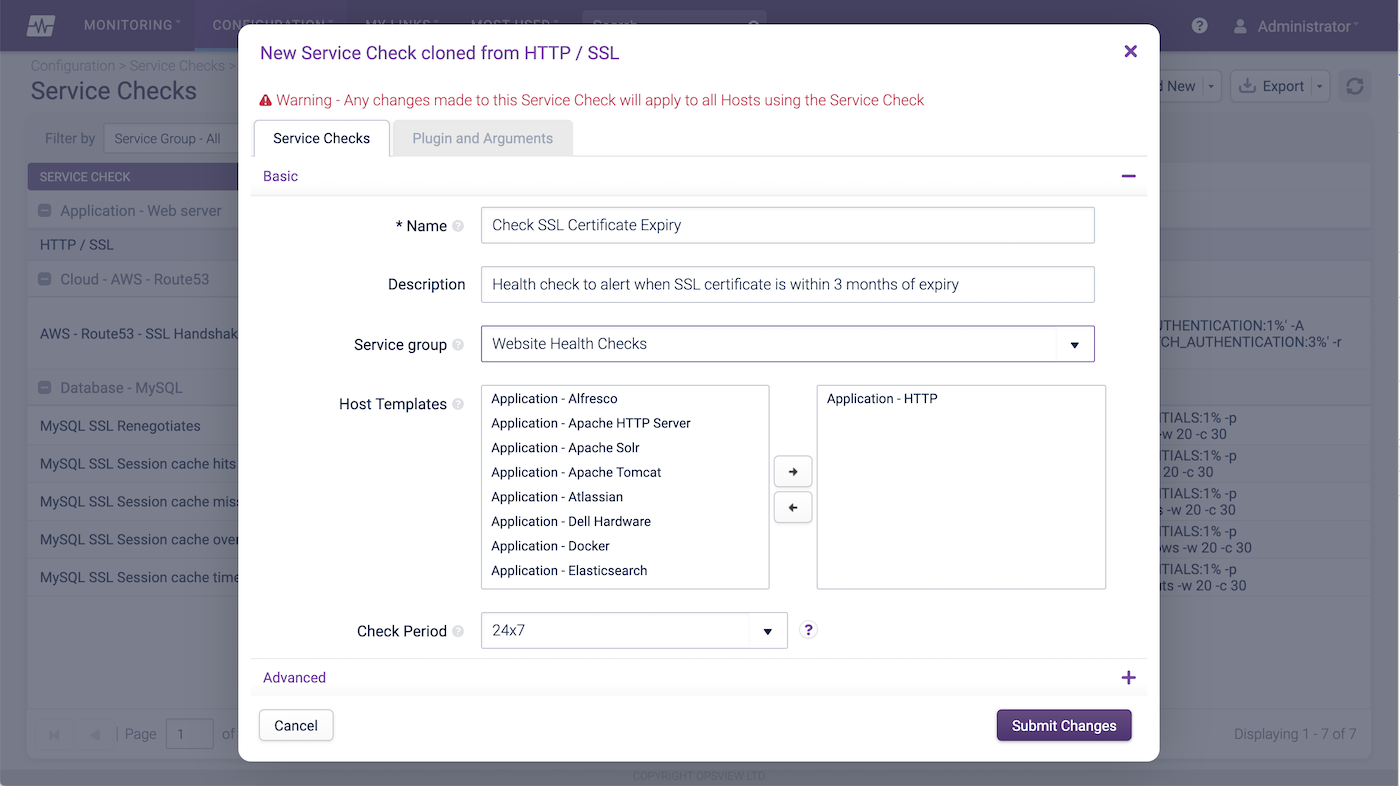This is a detailed description of a screenshot featuring a pop-up menu on the website MonitoringTM. The white square pop-up menu is centrally positioned on the screen, and a grey filter is applied to the background, which encompasses both the left and right sides of the pop-up menu, creating contrast and drawing attention to the menu.

The pop-up menu is the focal point of this screenshot. In the upper left corner of the pop-up, the text "It says," is displayed in blue font. Below it, the phrase "It says," is written again, but this time in red font. The pop-up contains two tabs near the top: "Service Checks" and "Plugins and Arguments," with "Service Checks" currently selected.

Beneath the selected tab, "Basic" is displayed in blue font, followed by several settings. The first setting is labeled "Name," with "Check SSL Certificate Entry Expiry" written next to it. Below this setting is a description: "Health Check to alert when SSL certificate is within three months of expiry." Further down, the setting "Service Group" is shown, categorized under "Website Health Checks."